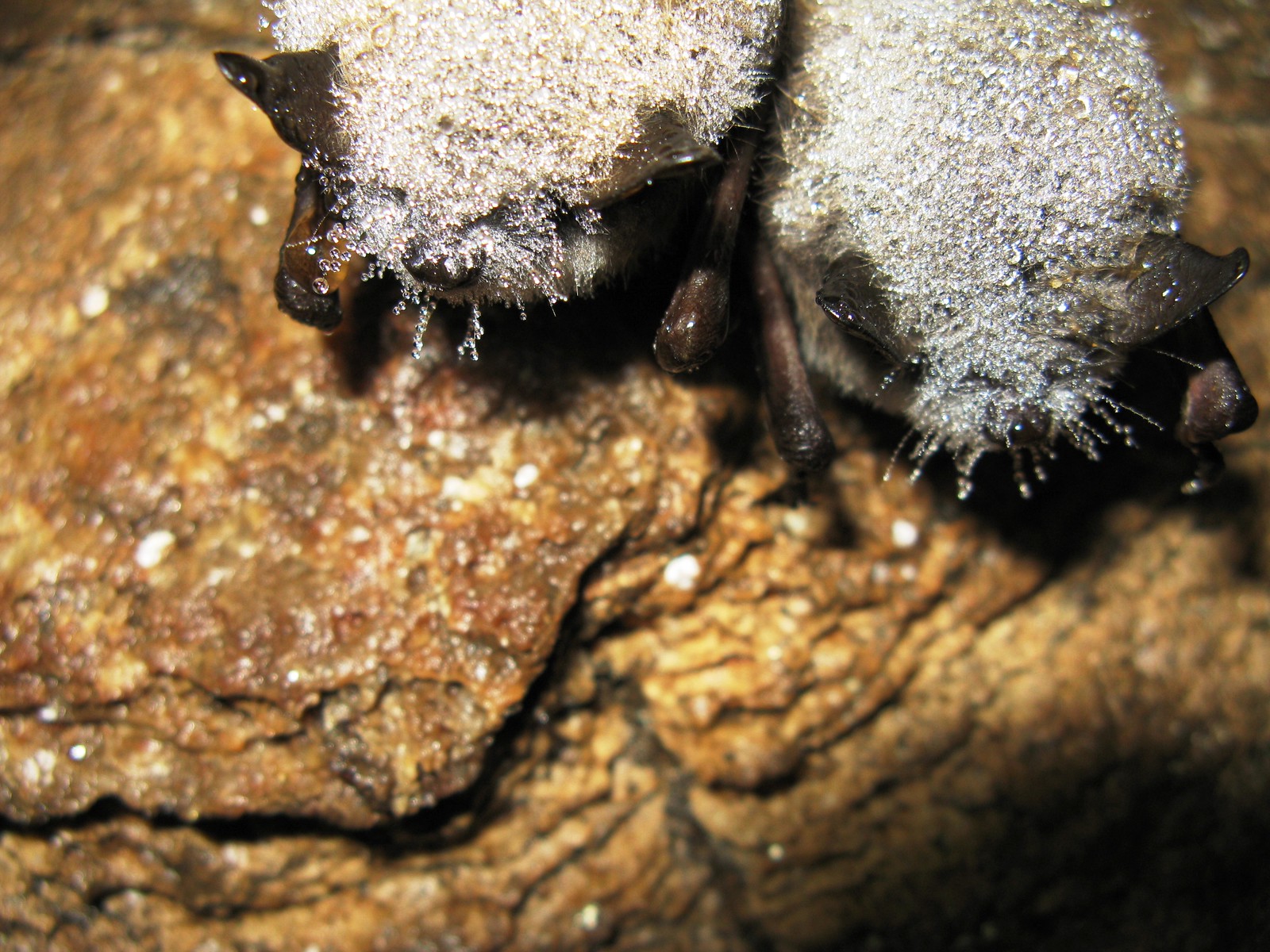The image depicts a dark cave, with a rocky, potentially wet surface taking up most of the frame. Toward the top of the image, there's an object that might be an animal, possibly bats, covered in a white coating, or it could be ice crystals forming on leaves. The cave features a variety of colors, including shades of gold, brown, white, black, and gray, and the rock surface has amber-like spots. The object in question appears to have dark brown areas that could resemble eyes. The overall setting is outdoors, though the exact time of day is unclear, and the scene is illuminated in such a way that highlights the gold and yellow tones, creating a slightly sparkling effect.